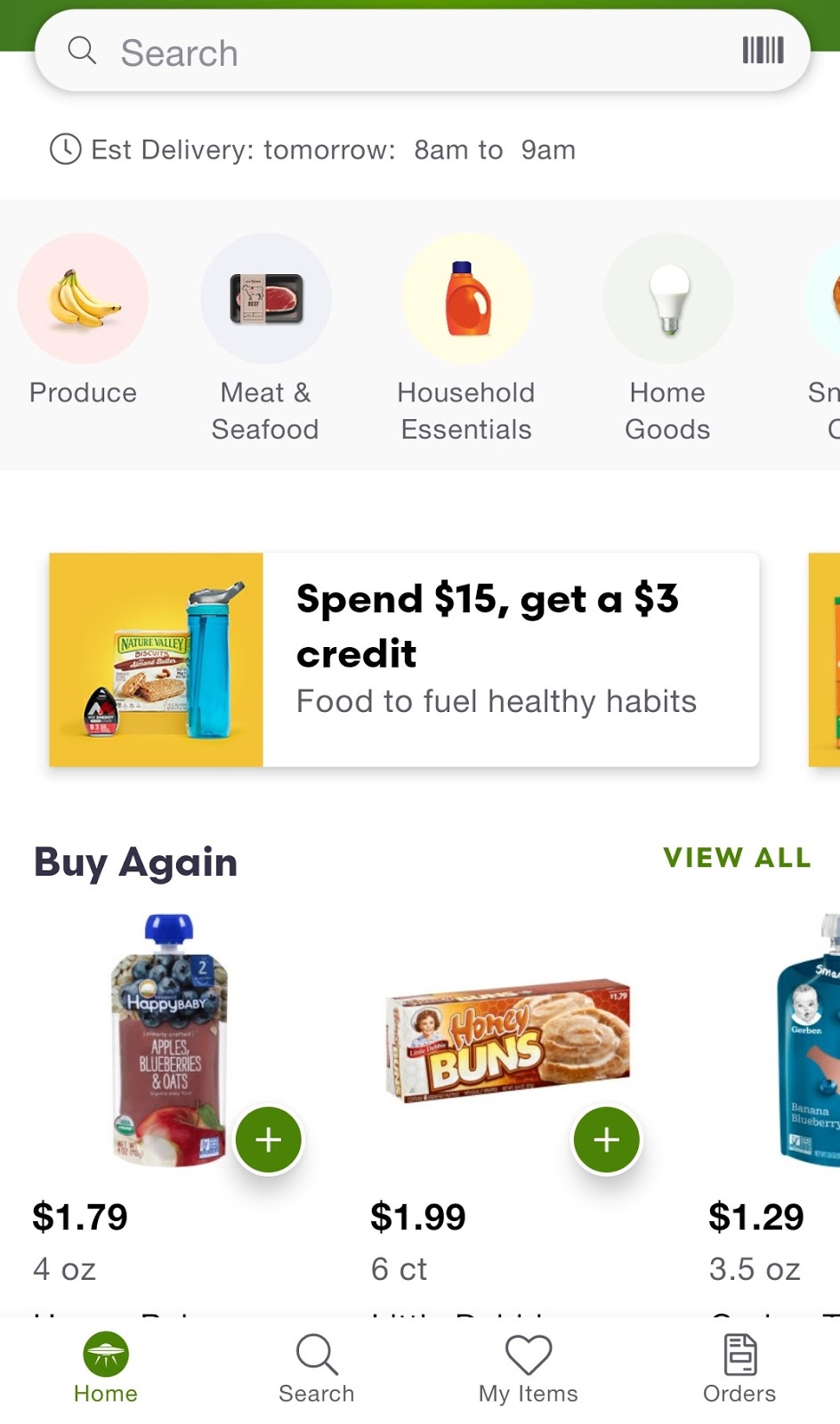The image is a screenshot, likely from a mobile phone, showcasing the interface of a shopping app, possibly Instacart or a similar grocery delivery service. At the top of the screen, there is a prominent green rectangle followed by a white circular search bar. Below the search bar, there's a white background displaying a message that reads, "Estimated deliveries tomorrow 8 a.m. to 9 a.m."

The app's main navigation is represented by a light gray bar with four circular icons. The first icon depicts bananas and is labeled "Produce." The second icon shows a tray of meat and is labeled "Meat & Seafood." The third icon, which displays a bottle of laundry detergent, is labeled "Household Essentials." The fourth and final icon features a light bulb and is labeled "Home Goods."

Beneath this navigation bar, there is a rectangular advertisement with a yellow background. The left side of the ad features an image, and to the right, there's text stating, "Spend $15, get a $3 credit. Food to fuel healthy habits."

Further down, the screen displays three square product images, though the rightmost image is partially cut off. The first product appears to be a small container of applesauce, priced at $1.79, with a green plus sign inside a circle next to it for adding the item to the cart. The second product is a six-count pack of Little Debbie Honey Buns, priced at $1.99. The third product, which is partially obscured, appears to be a blue bottle.